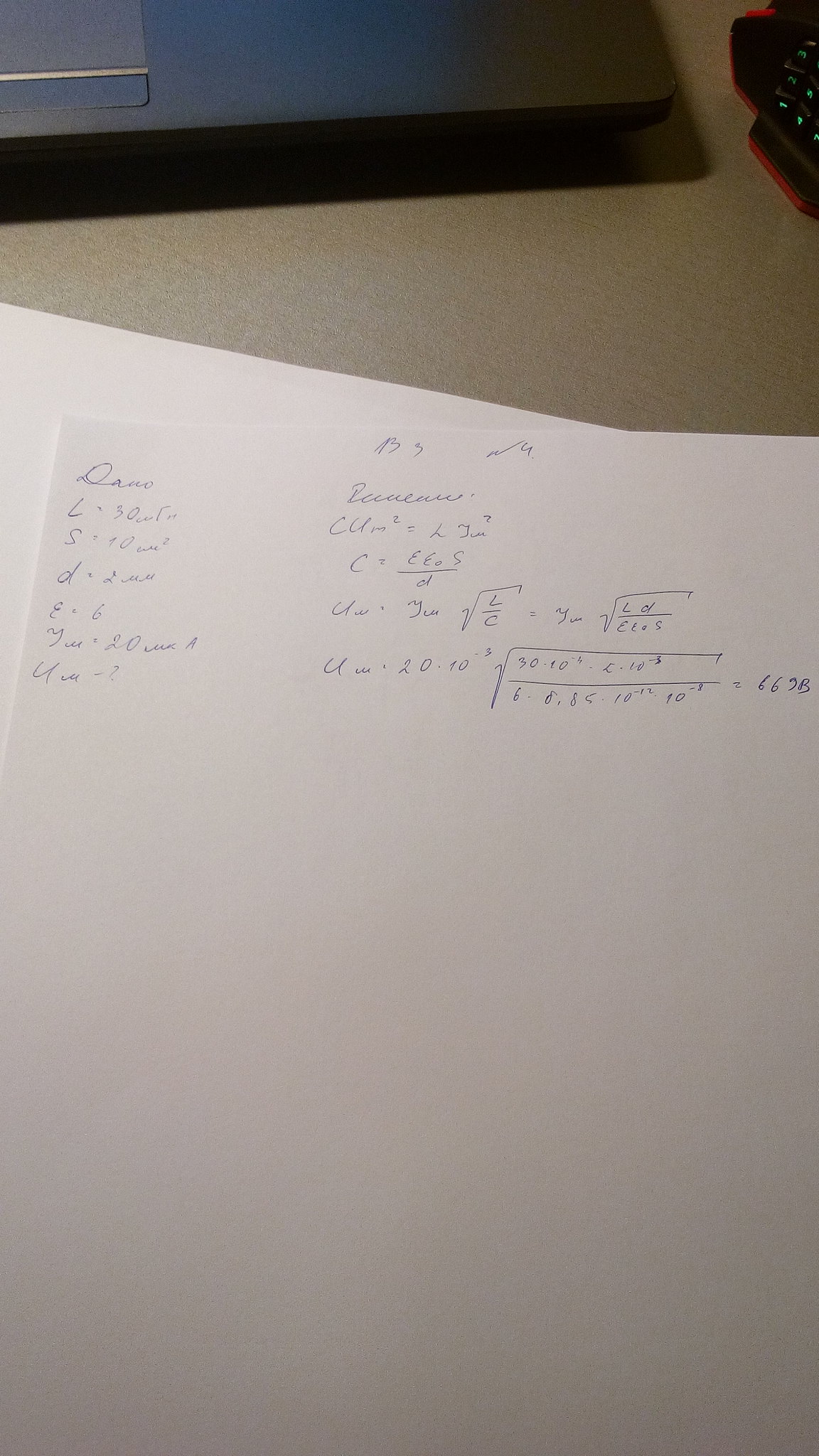The photograph captures a cluttered workspace featuring a handwritten math note on a piece of plain white computer paper, which is laid out on a table. The bottom half of a sleek, modern laptop with green backlit keys is partially visible in the upper right corner, slightly pushed aside to make room for the notes. The paper is sparsely filled with equations and statements written in blue ink, showcasing personal and somewhat difficult-to-decipher handwriting.

On the left side of the paper, several variables and equations are noted: 
- "Dano, L = 30"
- "W something M"
- "S = 10"
- "W to the second"
- "D = 2"
- "UU, E = 6"
- "YU = 20"
- "A, UU = ?"

On the right-hand side, additional mathematical expressions and shorthand notations include: 
- "B 3 WU"
- "because CUM to the second = LJU to the second"
- "C = EEOS/D"
- "UU = YU"
- "square root of L/C = YU square root of LD/EEOS"

These scribbled notes suggest an intricate problem-solving process, perhaps related to a college-level mathematics or engineering course. The overall scene conveys a diligent and focused effort to comprehend complex equations, set within a modern yet somewhat disorganized study environment.